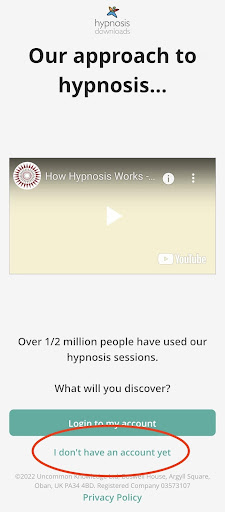The website displays a sleek and modern design with a light gray taupe background. In the center, there's an abstract graphic of a person, characterized by a circular head and stick-like limbs. The figure's legs are both blue, while the arms differ in color, with the left being red and the right yellow. Directly beneath this illustration, a bold and large heading reads "Our Approach to Hypnosis…" with an emphasis on the first letter "O" capitalized.

Below this, a prominent yellow rectangle catches the eye, featuring a burgundy circular graphic emitting rays. This graphic is accompanied by the text "How Hypnosis Works." Within this section, there's a white circle containing an "i" at the top, followed by three vertically aligned dots, indicating an interactive element, likely a video. The prompt allows playback through YouTube, as indicated by the logo, with engaging text that reads, "Over half a million people have used our hypnosis sessions. What will you discover?"

Towards the bottom, a greenish-blue tab stands out with the option "Log into my account" displayed in white text. Adjacent to it is a phrase, "I don't have an account," in matching blue text, encircled by a red oval. Finally, the "Privacy Policy" link is also present, ensuring easy access to important user information.